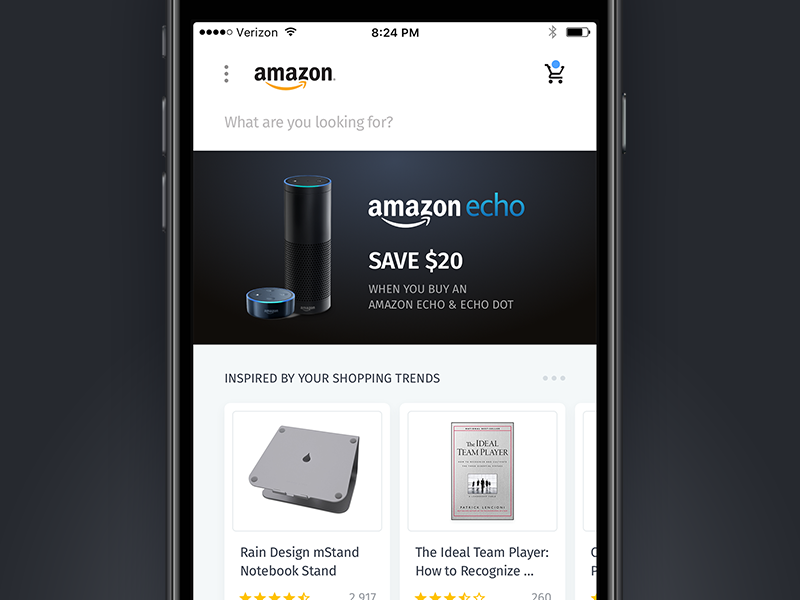In this image, a smartphone screen is prominently displayed, open to a web page on Amazon. The Amazon logo, characterized by the word "Amazon" in black text accompanied by a yellow arrow forming a smiley face, is located in the top left corner. Adjacent to this logo, in the top right corner, is a shopping cart icon with a blue circle, signaling the checkout button. At the very top center of the screen, the time is shown as 8:24 p.m.

The main portion of the screen features a vibrant banner advertisement for the Amazon Echo, a cylindrical, black smart speaker. The banner promotes a $20 discount when purchasing both an Amazon Echo and an Echo Dot. Below this banner, the page showcases a few products with customer ratings, including a notebook stand and a book titled "The Ideal Team Player."